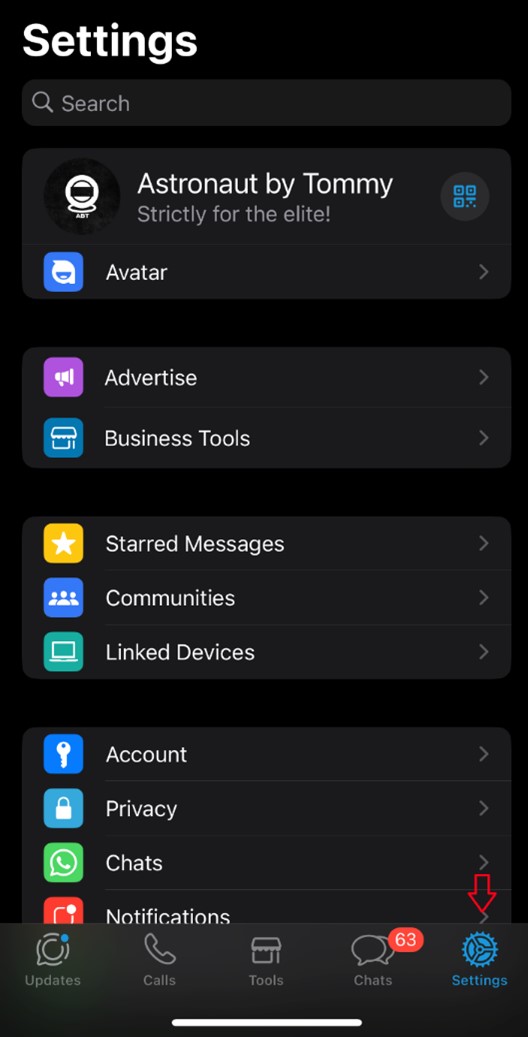The image is a heavily detailed interface layout featuring various icons and sections, predominantly integrating a dark theme. The top left corner features a white section labeled "Settings" and "Search" alongside a circular icon. Below this, there's text stating "Astronaut by Tommy," designated "strictly for the elite," accompanied by a QR code. 

To the right, there is an avatar and a purple circle labeled "Advertised." Nearby, a blue square titled "Business Tools" stands out, followed by a white/yellow square with a white star inside, presumably for "Star Messages." Additional options include "Communities" and "Link Devices."

Further down, there is a black space, and nearby, a blue square with a key icon, labeled "Account." Another blue square featuring an unlocked key icon represents "Privacy." Adjacent to these, there's a green square associated with "Chats" and a red square for "Notifications." Below that, a red down arrow points towards another section labeled "Updates," "Calls," "Tools," and "Chats," with a count of 63 notifications.

At the bottom, there's a white bar and a gray rectangle housing five icons. The settings section consists of ten distinct icons. This setup forms an intricate and organized user interface, likely for managing various account and application settings.